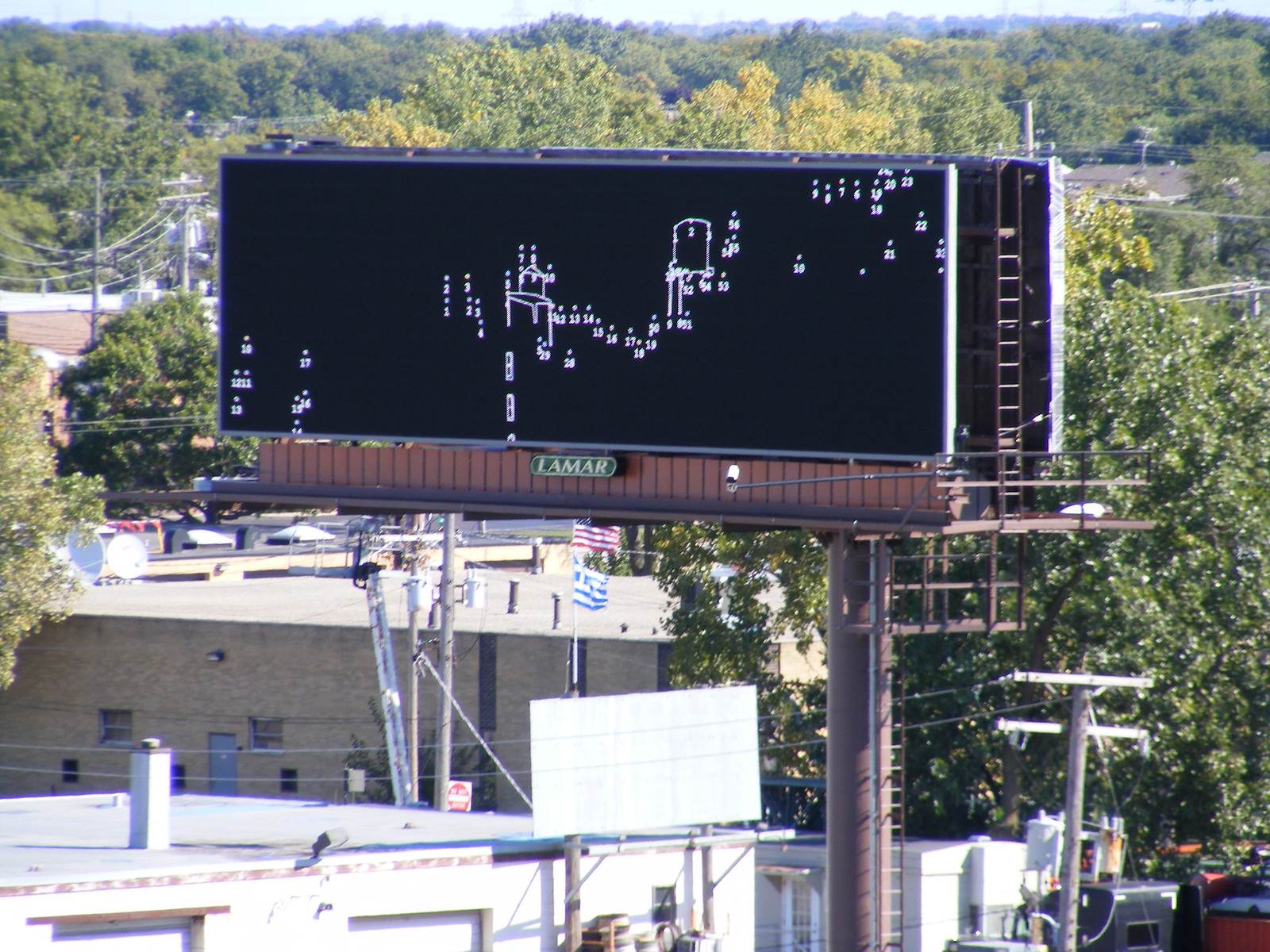The photograph captures an outdoor scene dominated by a rich array of tall trees with a blend of green, yellow, and brown foliage, set against a backdrop of a blue sky with some clouds and a faint skyline. There is a darker mountainous area in the distance. Numerous powerlines and telephone poles crisscross the image. In the foreground, several large buildings and businesses are evident, surrounded by the trees. One prominent building has a flagpole displaying an American flag and a blue flag with a white cross in the top left corner. A vehicle is parked in the bottom right corner of the image. Dominating the scene is a large steel billboard painted brown, featuring a black rectangular section with an erratic pattern of white dots, lines, and numbers, possibly resembling schematics or a draw-by-number design. The billboard's owner, "Lamar," is indicated in green letters within a green box. A ladder extends up the side of the billboard, suggesting maintenance access.